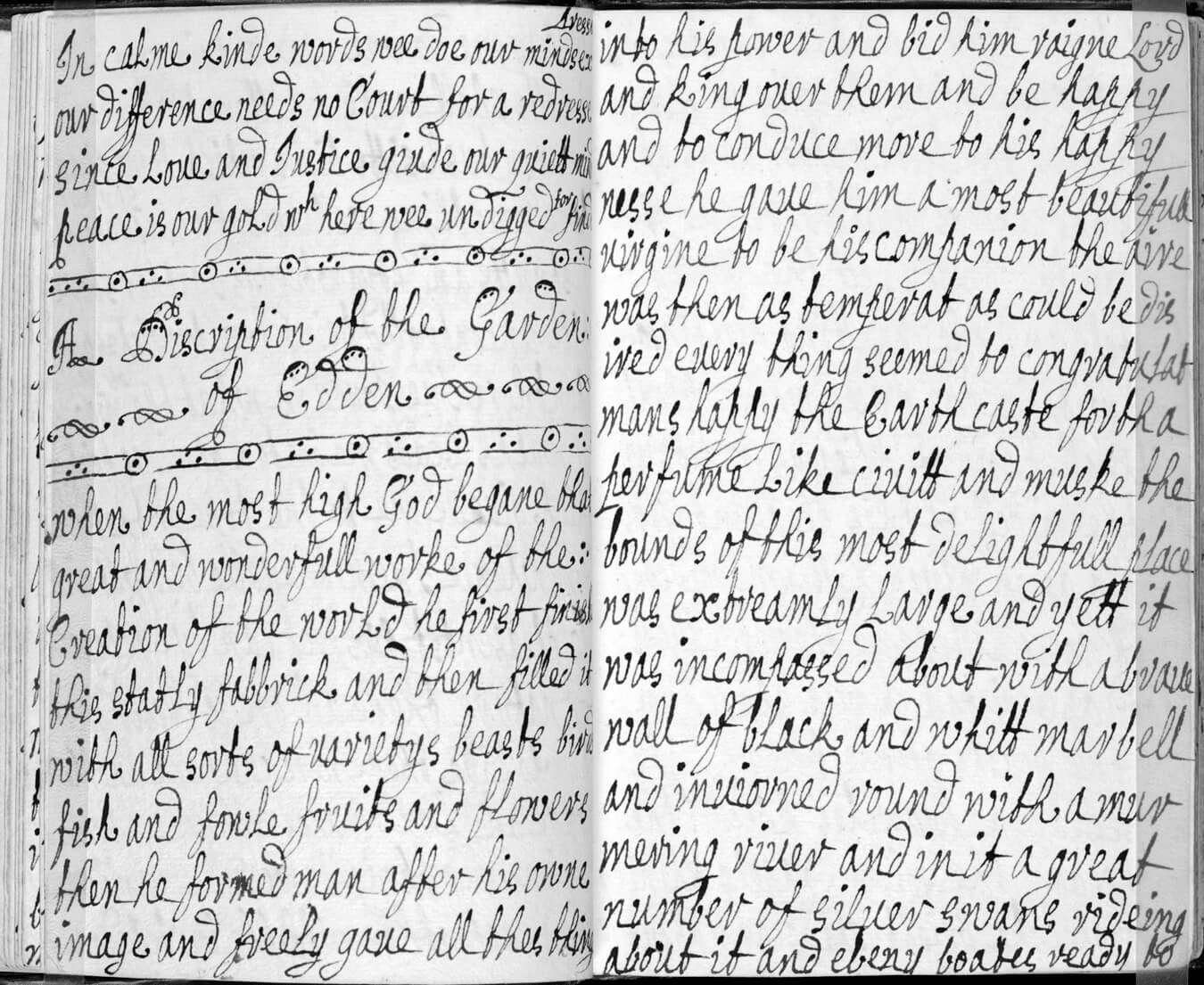The image features an open book with pages filled with long, narrow, handwritten cursive in black ink against a white background. Both the left and right pages are densely covered in this cursive writing, which spans from the very left to the very right side of each page. Midway down the left page, enclosed in a decorative black-lined box, is the title "A Description of the Garden of Eden." The cursive text is detailed but quite hard to read, consisting of calm, kind words that flow horizontally across the pages. The writing style appears quite novelistic and may be of religious nature, given the title and its connotations.